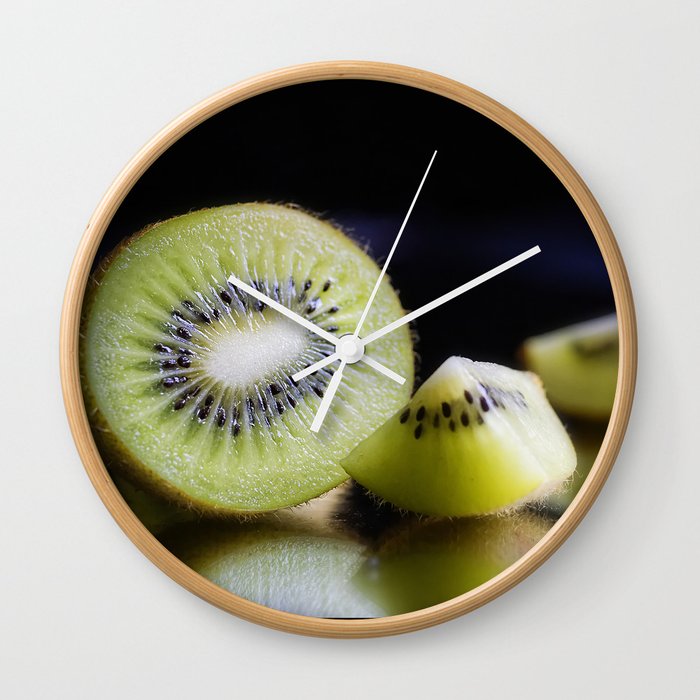This square, photoshopped image showcases a uniquely designed clock with a kiwi fruit theme. The circular clock face is crafted from a close-up photograph of several kiwi fruits, meticulously overlaid onto a round wooden frame. A small gap at the bottom edge reveals the composite nature of the image. The clock features white hour, minute, and second hands positioned at the center. 

Dominating the left portion of the clock face is a large, detailed slice of kiwi. Adjacent to this is another piece of kiwi fruit towards the right, while a slightly out-of-focus kiwi is positioned at the 3 o'clock mark. The kiwi fruits are depicted with intricate textures, showing their fuzzy exteriors and vibrant interiors marked by light green flesh and contrasting black seeds. 

The image is playfully lit, creating numerous shadows and highlights that add depth and realism to the kiwi fruits. The background of the clock face is a deep, jet black with a subtle blue tint, which adds contrast to the vivid green kiwis. This entire composition rests against a plain, very light gray backdrop, further emphasizing the clock's creative design.